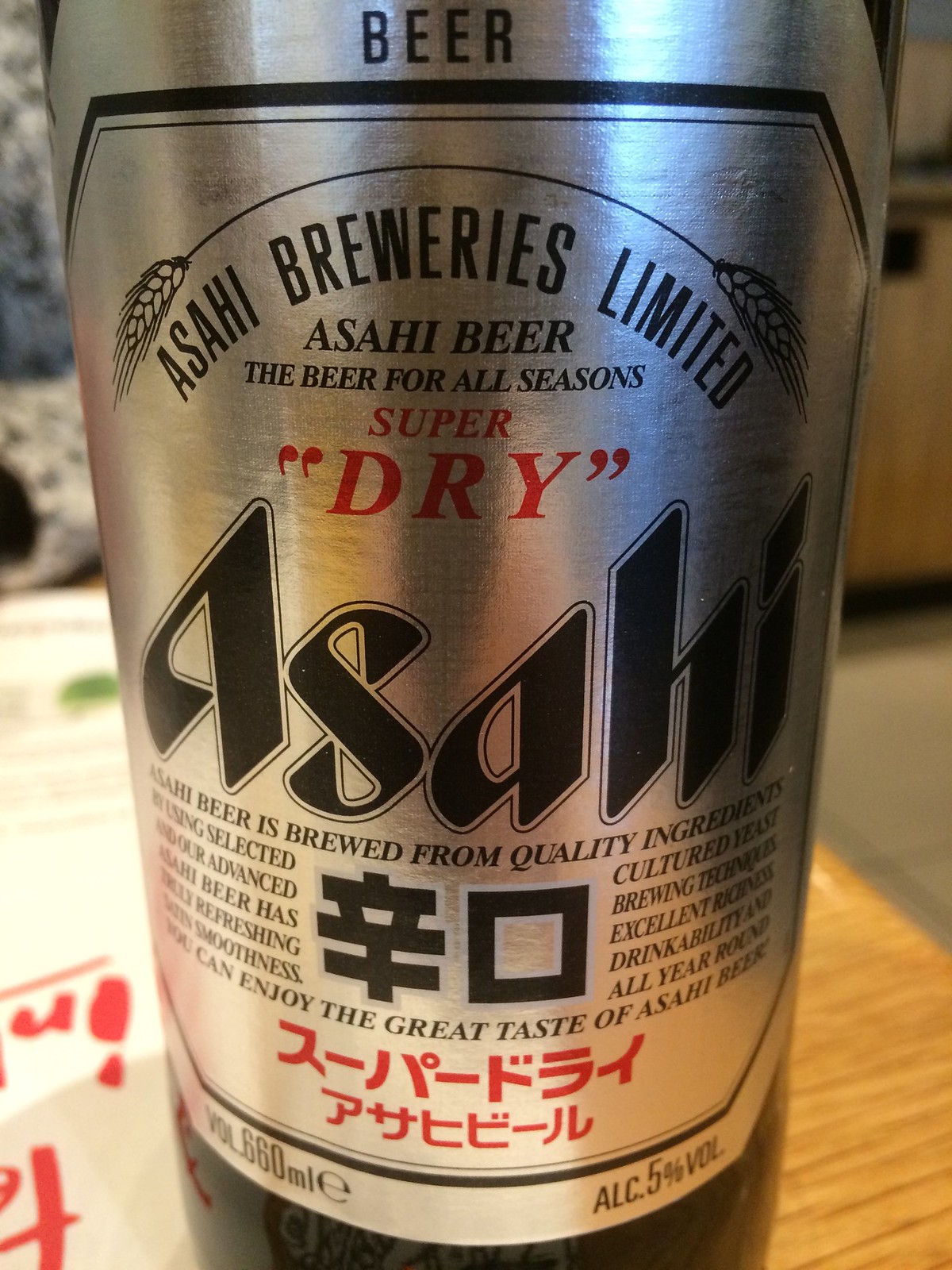This image features a close-up of a shiny silver can of Asahi beer from Asahi Breweries Limited, prominently placed on a light wood table. The beer can showcases numerous details including the text “Asahi Beer” and the tagline “Super Dry” in red. The label is adorned with various Japanese characters in black and red, underscoring its cultural origin. The description on the can highlights the quality and character of the beer, emphasizing it is brewed from quality ingredients using selected cultured yeast and advanced brewing techniques to offer excellent richness, refreshing drinkability, and smoothness all year round. Specification details are also included on the label, which states an alcohol content of 5% by volume and a total volume of 660 milliliters. Also visible in the image is a piece of white paper with red writing, placed underneath the beer can, although the text appears partly obscured and might be in Japanese.